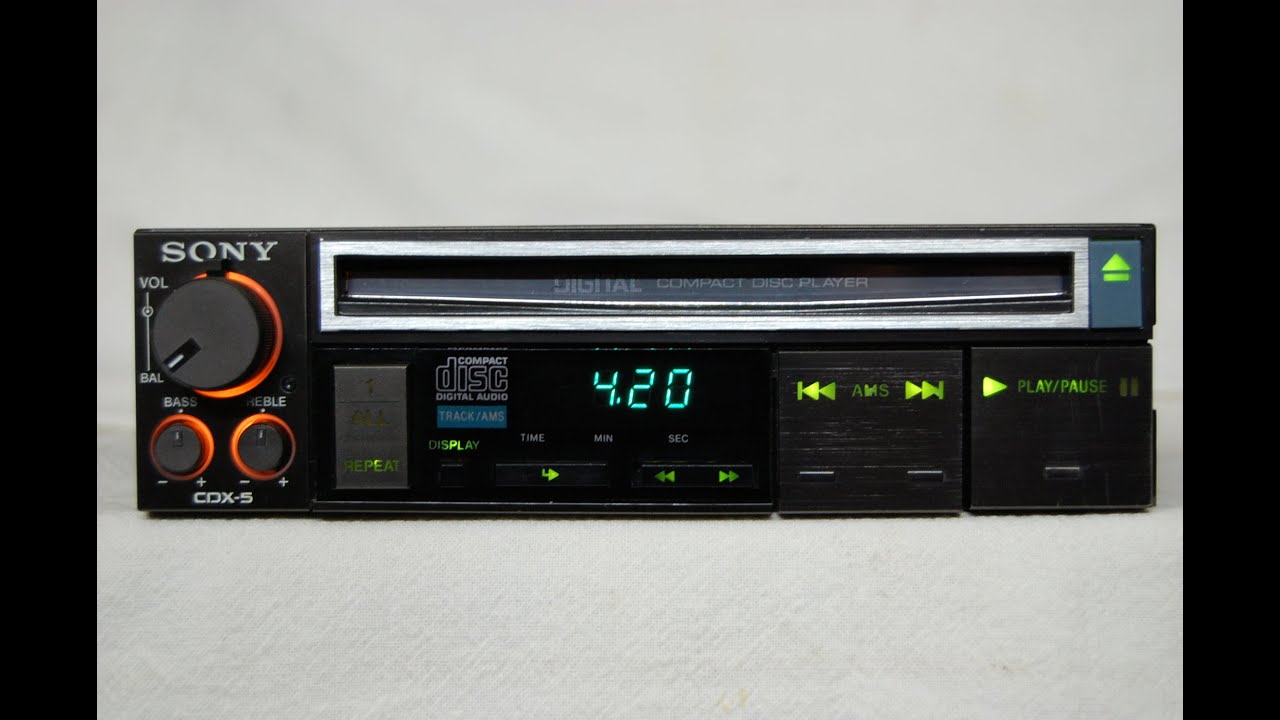The photograph depicts an old black car stereo system, rectangular in shape, with a small black border along its vertical edges and a light gray background. Prominently displayed on the top left corner of the stereo is the word "Sony" in white text. Below this, there is a large black volume knob encircled by an orange background, with the label "volume" next to it. Beneath the volume knob, there are two smaller knobs; the left one is labeled "bass" and the right one "treble." Further down, “CDX-5” is also inscribed in white text.

In the middle to the top right section of the stereo, there is a slot for inserting CDs. Surrounding the main interface, numerous buttons, illuminated in green, control various features including fast forward, rewind, play, pause, and enter. Some buttons display additional functions such as repeat, AM, display time, minute, and second. A blue LED display on the stereo shows the number "4.20". The stereo's branding is reinforced with "Compact Digital Audio Track / AMS" inscribed towards the bottom middle section.